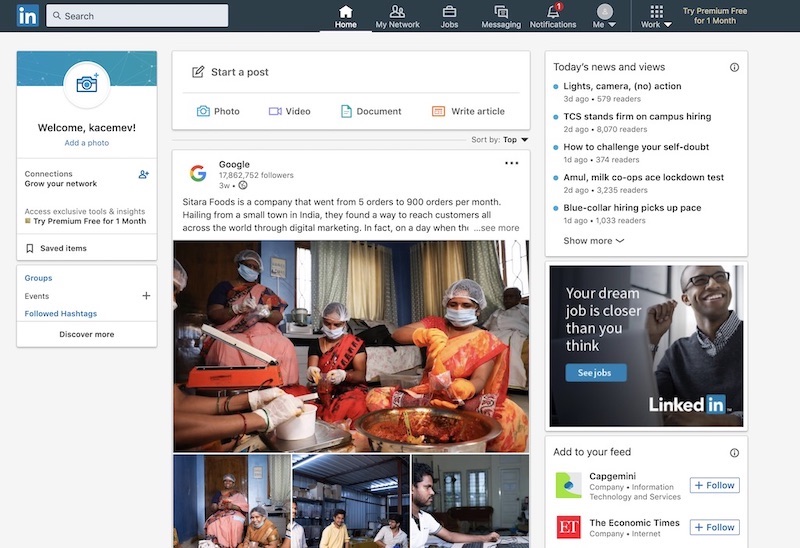This image shows a detailed view of a LinkedIn web page. In the upper left-hand corner, the iconic LinkedIn logo is prominently displayed, situated within the top navigation bar that spans the width of the page. To the right of the logo, a search bar is positioned, ready for queries.

Adjacent to the search bar are various menu options lined up sequentially from left to right: "Home," "My Network," "Jobs," "Messaging," and "Notifications," with the notifications icon indicating one new alert. Moving further along the menu bar, there is a profile icon labeled "Me," complete with a drop-down arrow for additional options. Another section is marked "Work," also accompanied by a drop-down arrow, indicating more functionalities. Additionally, a banner encouraging users to "Try Premium Free for One Month" is visible.

The main content of the page welcomes a user with the handle "kacemev," punctuated with an exclamation mark, emphasizing the greeting. The layout and design are characteristic of LinkedIn’s user interface, delivering a clear, user-friendly navigation experience.